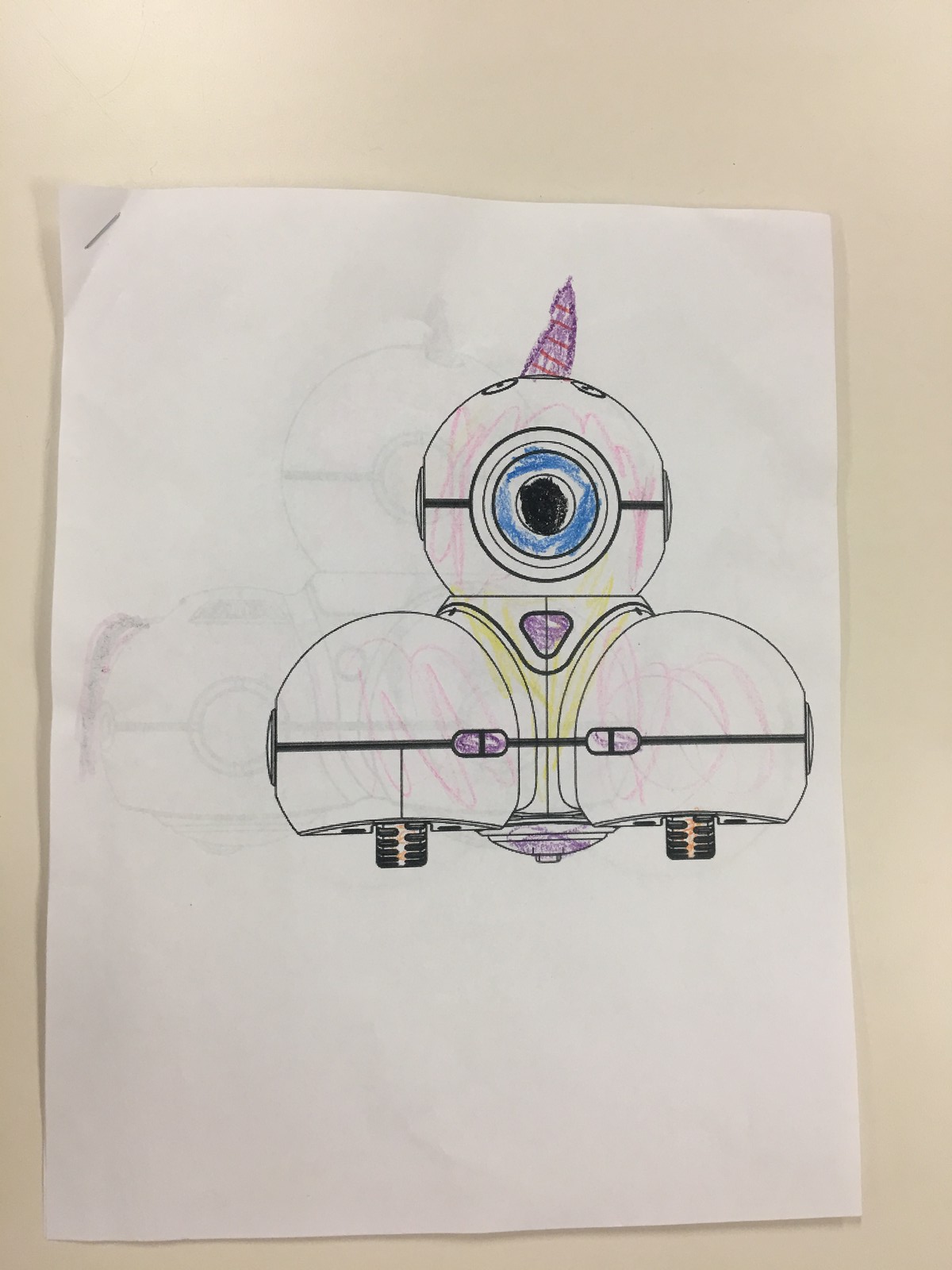This photograph showcases a completed coloring page, meticulously colored using a combination of crayons and colored pencils. The page, standard 8.5x11 inch printer paper, is secured by a staple in the top left corner. The image is set against a clean white background, possibly a tabletop or a bench. The central illustration features a futuristic robot with a unique design, characterized by two small treaded wheels on either side. Each wheel is encompassed by a large spherical hub. The robot's structure is a triangular arrangement of three spheres forming a pyramid shape. At the top of this pyramid sits a third sphere, distinguished by a prominent, large eye that gives the robot a watchful appearance. The careful coloring highlights the robot's contours and gives depth to its mechanical, yet whimsical design.